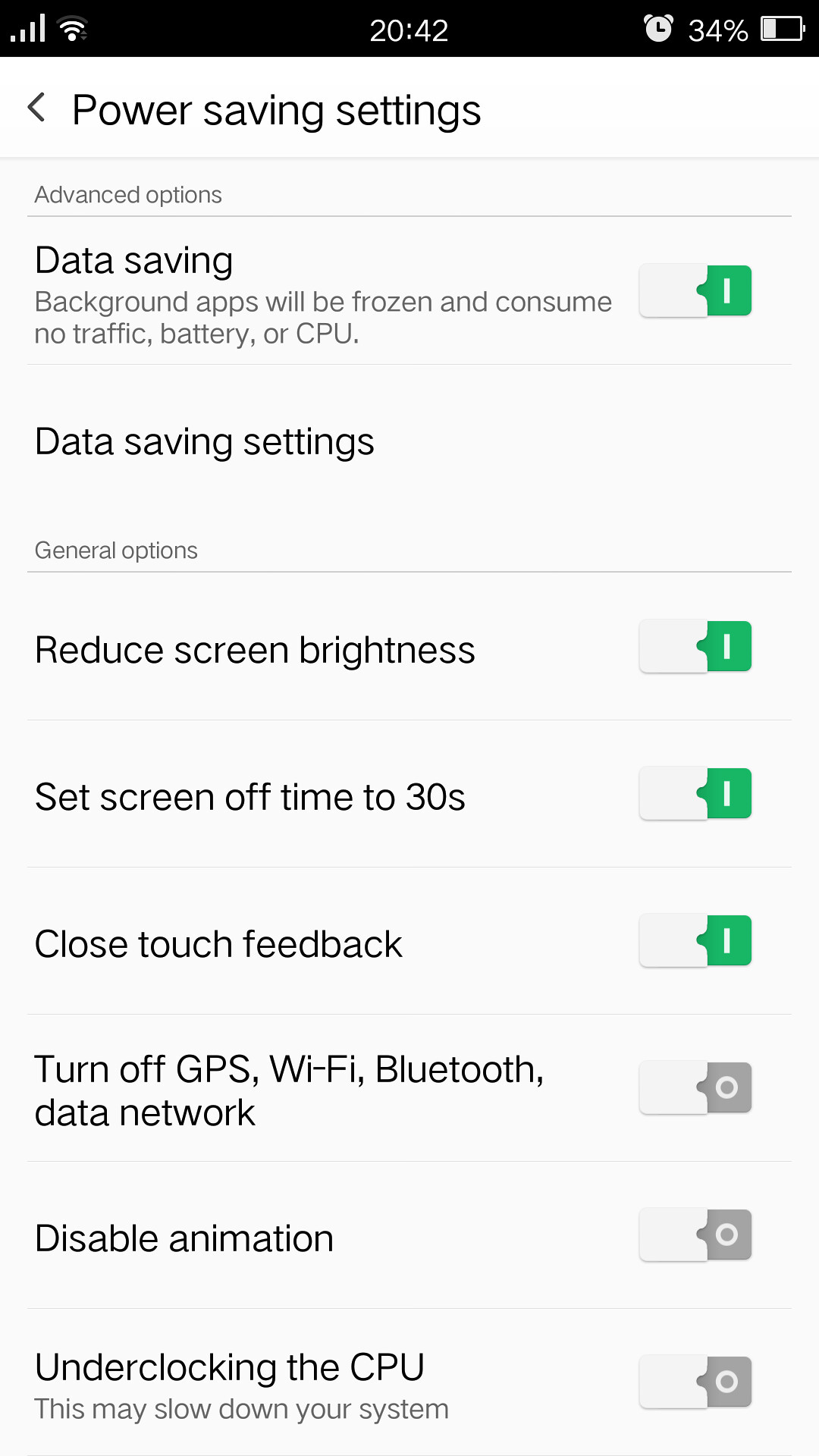A screenshot of device settings is displayed. At the top of the screen, the status bar indicates four signal bars, the time as 20:42, and the battery level at 34%. Below, the interface shows a section titled "Advanced Settings" with specific power-saving features. The descriptions mention that data saving and background apps will be frozen to prevent unnecessary use of traffic, battery, or CPU. The power-saving options include reducing screen brightness, setting the screen timeout to 30 seconds, disabling touch feedback, and turning off GPS, Wi-Fi, Bluetooth, and data network. Additionally, animations are disabled, and CPU usage is unlocked. Most of these options are toggled on, indicated by green switches, except for the last three options which are toggled off, shown with gray switches.